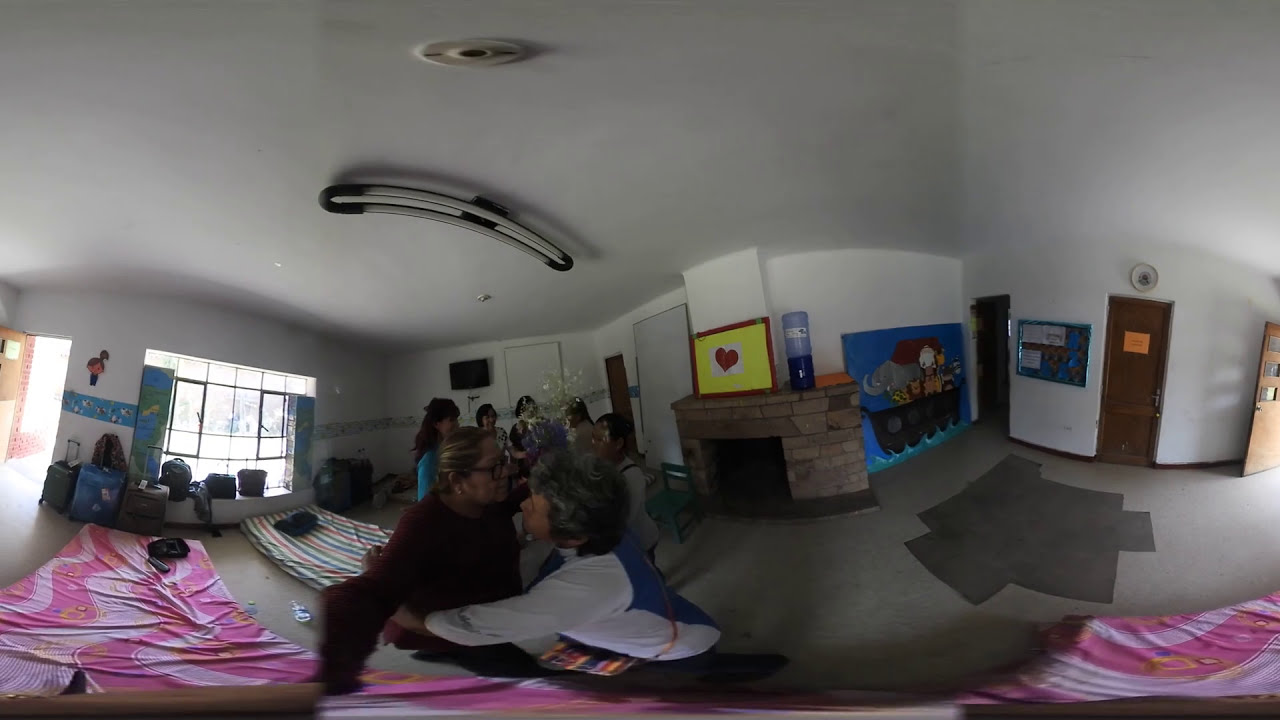The image depicts a 360-degree panoramic view of a room with white walls and a gray concrete floor. In the foreground, a man and a woman are seen embracing on what appears to be yoga mats or thin mattresses. Stretching across the floor is a long piece of pink and fuchsia fabric, and nearby, another person is lying down with someone possibly hugging them. The room features a large semi-open window to the left, flanked by an open doorway that leads outside. Against the left wall is a small stone fireplace with some artwork above it, including one piece with a yellow background and a red heart, and another depicting animals on a boat reminiscent of Noah's Ark. To the right of the fireplace, a door with a bulletin board can be seen. In the background, a group of people, predominantly women, are gathered and appear to be holding up a flower. The right side of the room features three doors, with the leftmost and rightmost doors open, and the middle wooden door having a clock above it. Additionally, some hand-drawn paintings, including a cartoon version of Noah's Ark, decorate the room, giving it a warm, communal ambiance.